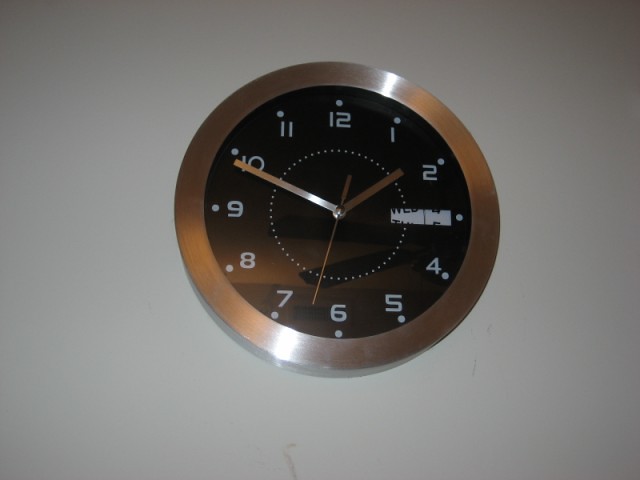This photograph captures a round wall clock mounted on an off-white, slightly grayish background. The clock boasts a sleek, silver metallic frame and features a black clock face adorned with striking white numerals. Three silvery hands—hour, minute, and second—point precisely, although they currently lie in between specific numbers. A unique aspect of the clock face is a cutout section designed to display the date, which, in this moment, is transitioning between two dates.

Several white polka dots strategically placed near the numerals and a white-dotted circle at the center add artistic details to the design. The clock face exhibits a subtle reflection of ambient light, accompanied by minor smudges, lending a touch of realism to the image. The photograph itself stands out for its excellent quality, presenting a crisp and clear depiction of this sophisticated timepiece.